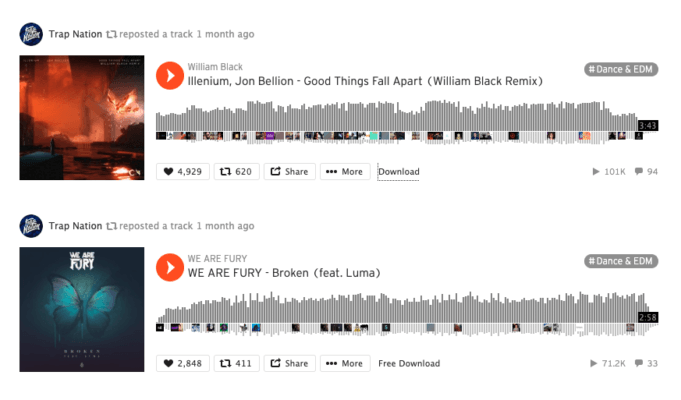The image features a clean white background, adorned with multiple sections of black text and colorful visuals. On the left side, a header reads, "Trap Nation reposted a track one month ago." Directly below this, there is a vibrant, color photograph that appears to depict a city scene with several explosions. Adjacent to this photograph on the left, an orange play button is positioned, followed by text that details the track information: "William Black, Illenium, Jon Bellion - Good Things Fall Apart (William Black Remix)." Additionally, the text includes hashtags "dance" and "EDM," further describing the music genre. The post has garnered 4,929 likes, 620 reposts, and offers several interactive options including a share button, a "more" button, and a download button. The track has been played 101,000 times and received 94 comments.

Below this section, the phrase "Trap Nation reposted a track one month ago" is reiterated. Following this, an image of a butterfly is placed, with white text above it reading "We Are Fury." To the right of this butterfly image, another orange play button is visible, accompanied by the text, "We Are Fury - We Are Fury Broken (featuring Luma)." The hashtags "dance" and "EDM" are included again for genre specification. This post has accumulated 2,848 likes and 411 reposts, along with options for sharing, more information, and downloading the track. This track has been played 71,200 times and has 33 comments.

The layout and organization of the various elements—text, images, buttons, and interactive features—create a structured and informative visual representation of the music reposts by Trap Nation.